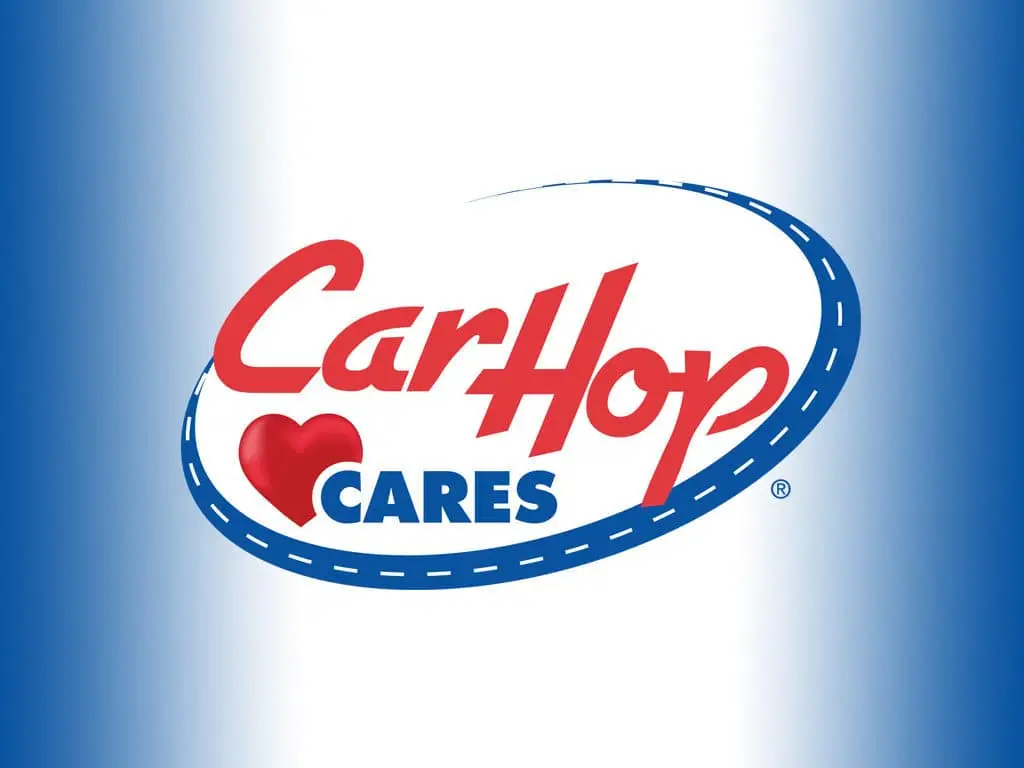The logo for Carhop features a sophisticated design with a dynamic color gradient background, transitioning from dark blue on the outer edges to bright white at the center. This gradient forms a visual effect of three horizontal stripes that seamlessly fade into one another. In the heart of the logo, an elongated oval shape, outlined by a blue border symbolizing a road with a white dashed line, frames the main elements. Bold red text prominently displays the company name "Carhop," characterized by a blend of block and cursive styles that give it a unique, stylized appearance. Directly beneath, in simple block letters, the slogan "CARES" is written in blue, underscored by a red heart symbol, emphasizing the company's commitment to care. A small encircled "R" at the bottom right denotes the trademark. This cohesive logo effectively conveys Carhop's brand identity and values, integrating both visual and textual messages.